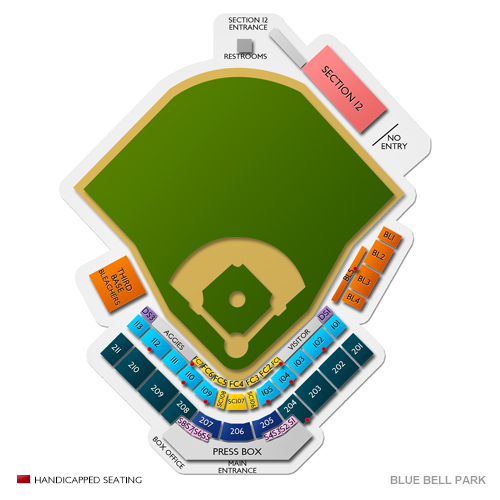The image features a detailed layout with various sections labeled. Against a white background, there is an entrance labeled "Section 12" near the restrooms. An oval shape is marked with "Section 12, No Entry." The building labels BL1 through BL5 are represented, with BL1 and BL5 marked by orange rectangles, and BL5 also featuring a red dot.

The seating arrangement includes blue squares representing sections 101 to 105 and sections 109 to 113. Notably, there are dots on sections 102, 104, 105, 109, 110, and 112. The third base bleachers are also indicated.

Additionally, more blue squares mark sections from 201 to 211, with a red circle highlighted on section 204. The layout specifies the press box and main entrance locations as well.